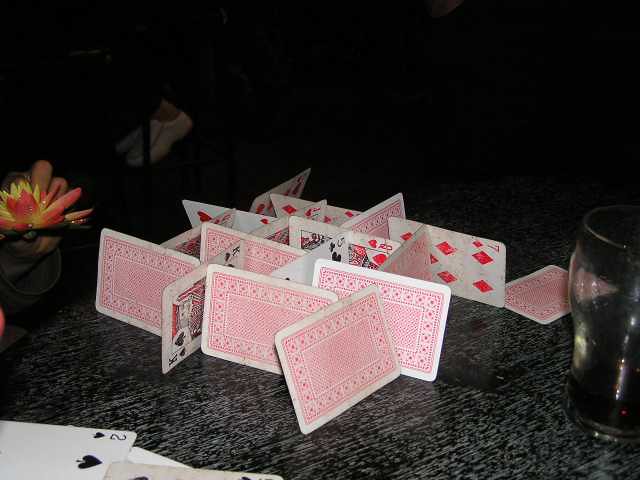The image captures a cluttered scene on a dark table with a black surface featuring white grain patterns. In the center, a precarious card tower is in the process of being built, with cards leaning against each other for support. Visible cards include the two of spades at the bottom, the king of spades, the five of clubs, the queen of hearts, and the seven of diamonds, along with other indistinct cards showing hearts and diamonds. 

To the left side of the image, a person's hand is holding a decorative lotus flower, adding an element of whimsy. Just above this hand, a shoe can be seen, suggesting the table is in close proximity to a seating area. Off to the right is a nearly empty glass, containing the remnants of a dark-colored beverage. The cards themselves appear old and worn, contributing to a sense of nostalgia. The overall scene suggests an ongoing card game or a creative attempt at building a card tower.